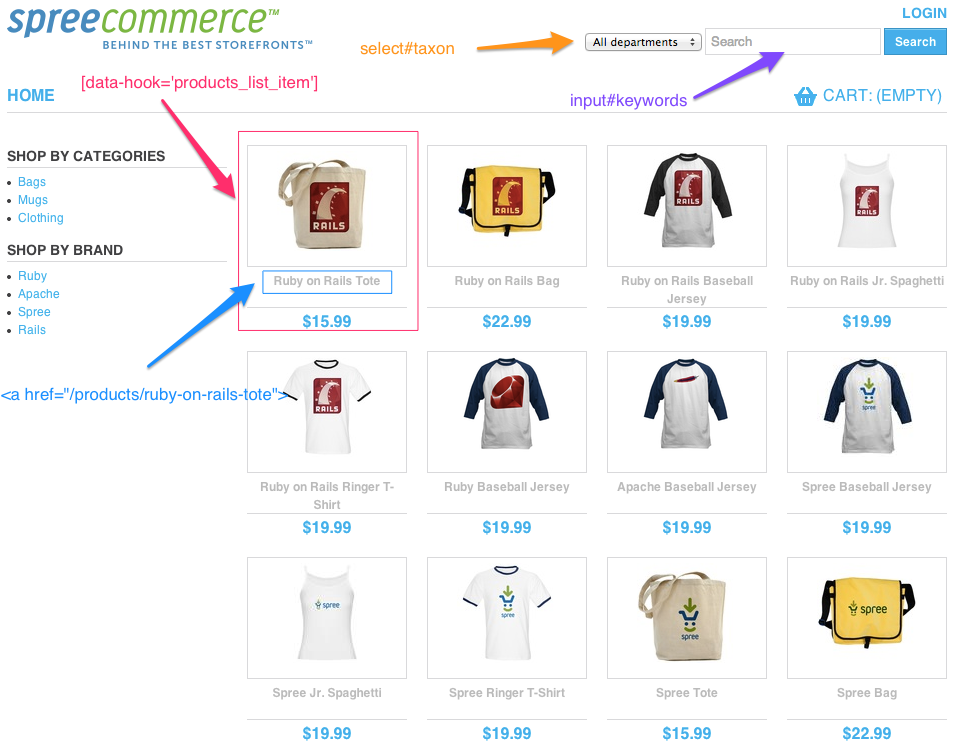The screenshot features an e-commerce website with a clean white background. On the left side of the page, the site branding is displayed with the text "Spree" in blue and "Commerce" in green, followed by the tagline "Behind the Best Storefronts" in blue font. Below this, there is a vertical navigation column. The top of this column lists "Home" in blue, followed by sections labeled in black as "Shop by Categories" and "Shop by Brand." The "Shop by Categories" section includes blue links for "Bags," "Mugs," and "Clothing," while the "Shop by Brand" section features blue links for "Ruby," "Apache," "Spree," and "Rails."

On the right side, the interface includes a drop-down menu labeled "All Departments," an empty search box, and a search button in blue. Above the search box, there is a blue "Login" button.

Below these elements, the main content area displays a grid of 12 square product images arranged in three rows and four columns. The showcased items include a tote bag, a messenger bag, a baseball tee, and a tank top. Each image has a price listed beneath in blue.

Several arrows on the page annotate different elements. A red arrow points to the product image grid, labeled "Data Hook Products." An orange arrow points to the "All Departments" drop-down menu with the label "Select Taxon." A blue arrow indicates the search bar with the label "Input Keywords," and a light blue arrow points to product names with the label "Ahref Products Ruby on Rails Tote."